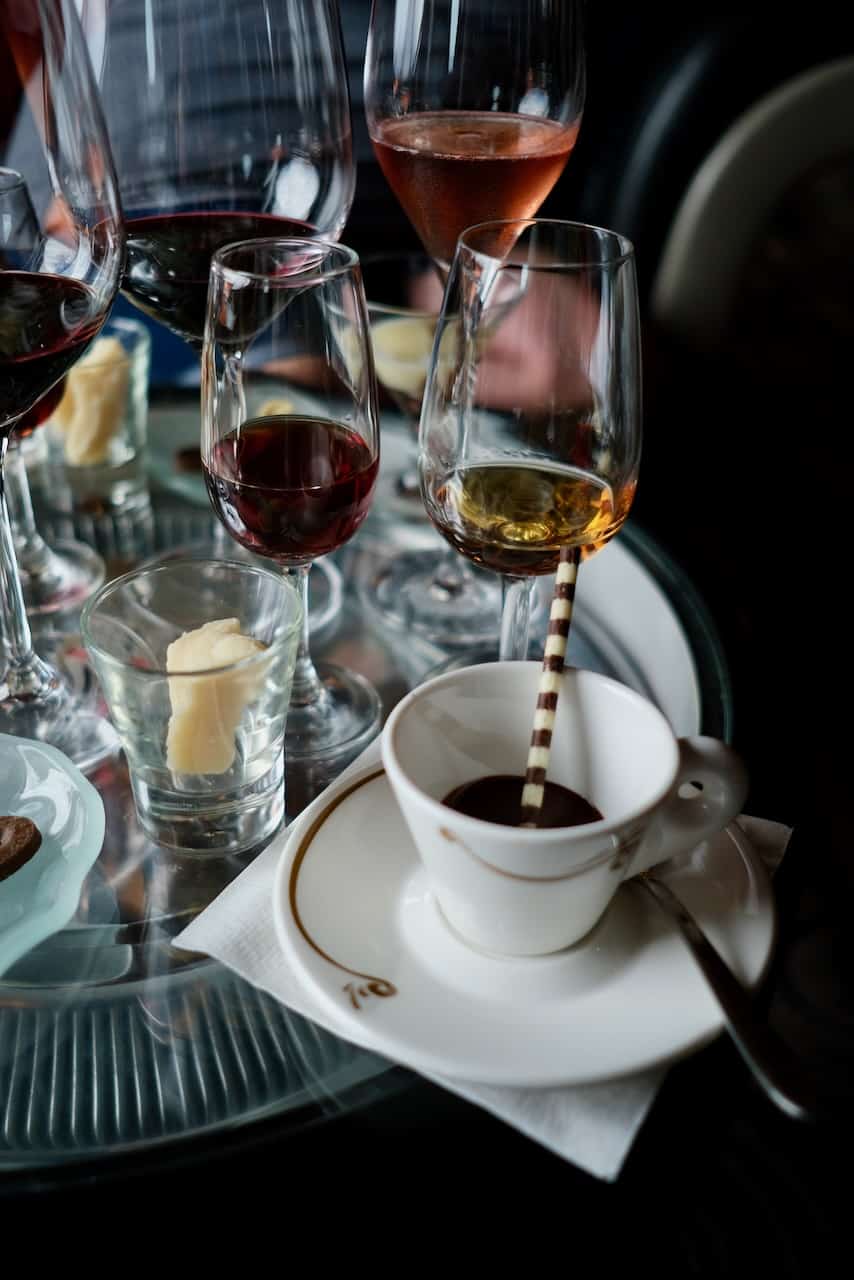The image captures the aftermath of a meal and drinking event, with a variety of glasses scattered on a tray or clear glass table. Centrally positioned is a white ceramic coffee cup with an ear, partly filled with a dark brown liquid, likely coffee or hot chocolate. Dipped into the cup is a brown and white-striped pirouette cookie. This cup rests on a white saucer adorned with a goldish-brown swirl, next to a silver spoon. Surrounding it, there are several wine glasses: two larger ones filled with red wine, a smaller wine glass holding a lighter-colored wine positioned beside them, and another glass with a low level of yellow liquid, possibly white wine. Additionally, there are two smaller glasses; one contains dark red wine, and the other holds a bubbly liquid, possibly beer or champagne. In the background are more wine glasses with varying contents, including a rosé and a burgundy-colored wine. The scene suggests the conclusion of a lively dinner party, now devoid of people.